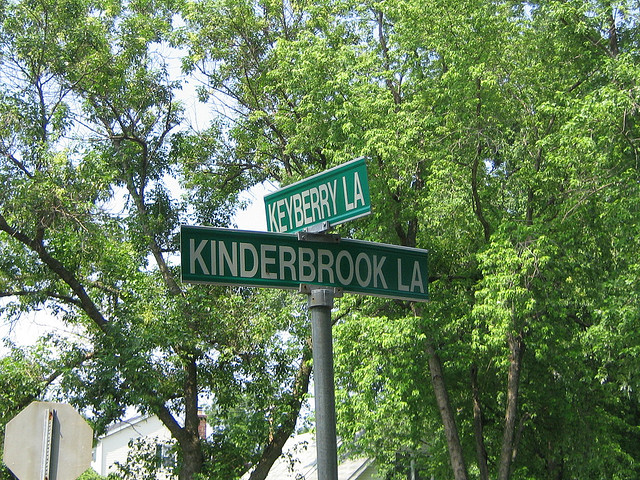This detailed photograph captures a sunny outdoor intersection within a leafy neighborhood. Dominating the scene are two green street signs with white lettering mounted perpendicularly atop a round gray steel pole. One sign reads "Kinderbrook Lane" while the other signifies "Keyberry Lane." The sunny backdrop features lush, green-leafed trees with sunlight filtering through, and beyond them, a glimpse of white residential houses, possibly hinting at a sloping landscape. Additionally, the bottom left corner reveals the white, metal-backed rear of a stop sign affixed to its post. The sky above is a vibrant blue with scattered, puffy clouds, enhancing the picturesque daytime ambiance.